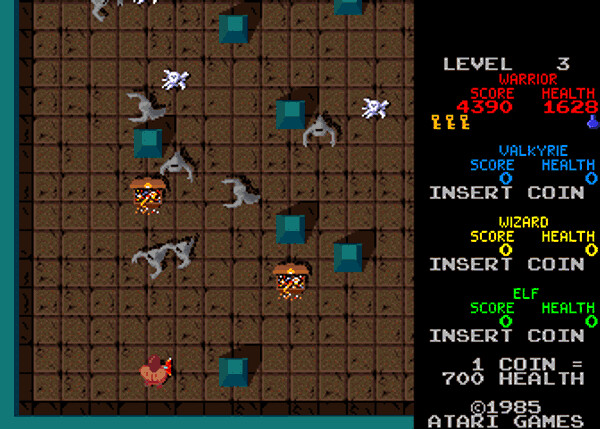A detailed caption for this image could be:

"A screenshot of a vintage 1985 Atari video game showcases a simple yet engaging design typical of older gaming graphics. The scene is set in a maze-like environment with various turquoise and aqua-colored cubes laid against a dark brown, tiled background. Amidst the maze, silver-gray creatures reminiscent of fish but equipped with large, powerful arms traverse the scene. Additional details include small pixelated images, such as a pile of bones topped with a skull, lending a sense of adventure and danger. On the right side of the image, a black background displays colored stats in red, blue, yellow, and green for different characters named Warrior, Valkyrie, Wizard, and Elf. The bottom of the screenshot bears a light gray copyright note stating '© 1985 Atari Games,' indicating the game's retro origins."